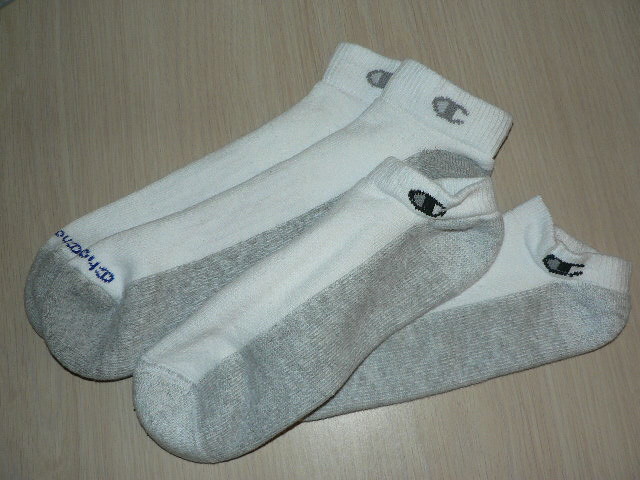This color photograph, taken indoors, features two pairs of Champion brand socks neatly placed on a hardwood floor. The background is a uniformly brown wooden surface, creating a simple, natural backdrop. Each pair of socks consists of gray bottoms and white tops, and both pairs appear to be new and clean. The larger pair, likely men's socks, are adorned with the word "Champion" written in blue across the toes and have the classic Champion logo in gray near the top of each sock. These socks are ankle-height. The smaller pair, which looks like women's or possibly children's socks, does not have any writing on them but still features the Champion logo. Both socks in this pair are also ankle-height. The photo's focus on the different sizes suggests a comparison between the two pairs.